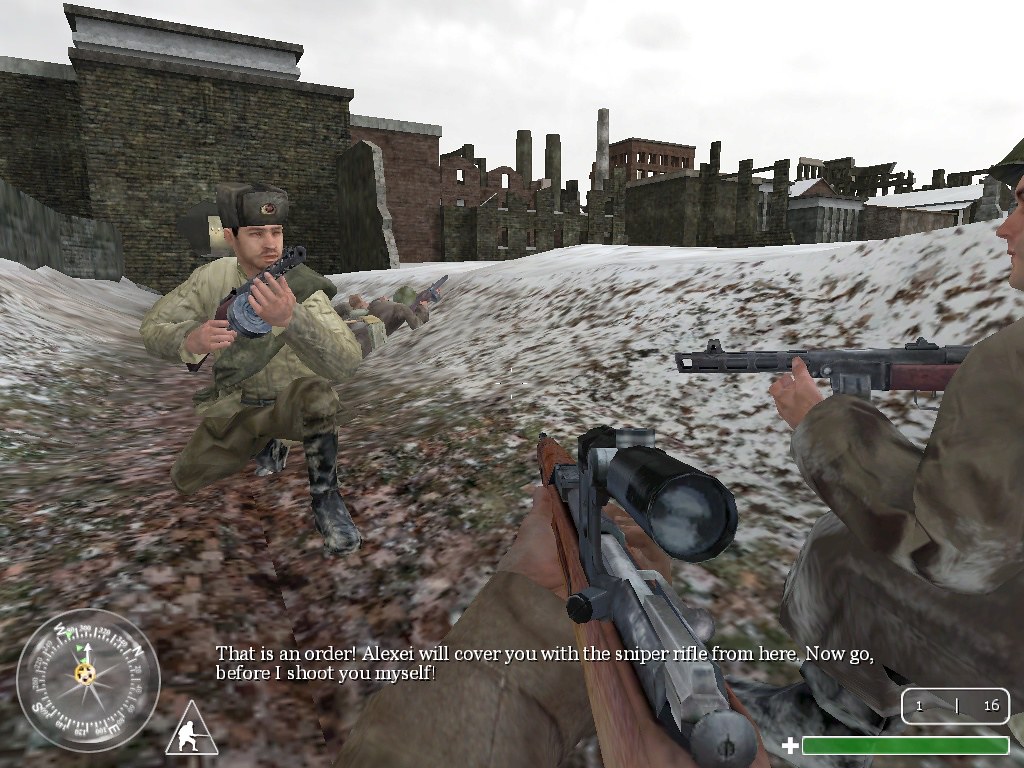In this scene from a video game, two characters, who appear to be Russian, are locked in a tense confrontation. One of them, named Alexey, is issuing a stern command to the other. Alexey declares that he will provide cover with a sniper rifle from their current position and warns that if they don't make a move, he'll handle it himself. The setting is an eerie, desolate area just outside a bombed-out and destroyed town. They are huddled together in a trench, lightly dusted with snow. The trench walls appear to be constructed from stone with concrete topping them off. The surrounding environment has the feel of an abandoned industrial site, with tall chimneys poking skyward from the derelict factories. Snow gently blankets the rooftops, adding a cold, bleak atmosphere to the scene. Despite the player's perspective focusing on one individual, the urgency and intensity suggest a bigger impending assault on the devastated town.